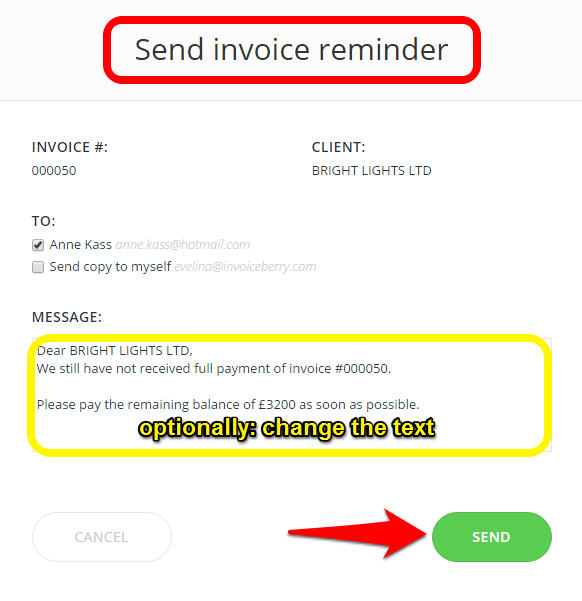The image displays an invoice reminder page designed for ease of understanding and action. At the top of the page, prominent black text reads "Send Invoice Reminder," framed by a red rectangular outline with rounded corners to highlight its importance. Below this, a gray line subtly separates the header from the content.

The content begins with "Invoice Number: 000050" on the left side, and "Client: Bright Lights LTD" on the right. Further down, it shows the recipient's information: "To: Anne Cass, Anne.Cass@hotmail.com." There is a checkbox labeled "Send copy to myself: Evelina at invoiceberry.com," which remains unchecked for this instance.

The message area contains a predefined note: "Dear Bright Lights LTD, we still have not received full payment of invoice number 000050. Please pay the remaining balance of £3,200 as soon as possible." This text is surrounded by a yellow outline with a black border, indicating that it can be optionally changed.

At the bottom of the page, two action buttons are available. On the bottom left, there's a "Cancel" button, while on the bottom right, there's a green "Send" button, accompanied by a large red arrow pointing to it, emphasizing the primary action of sending the reminder.